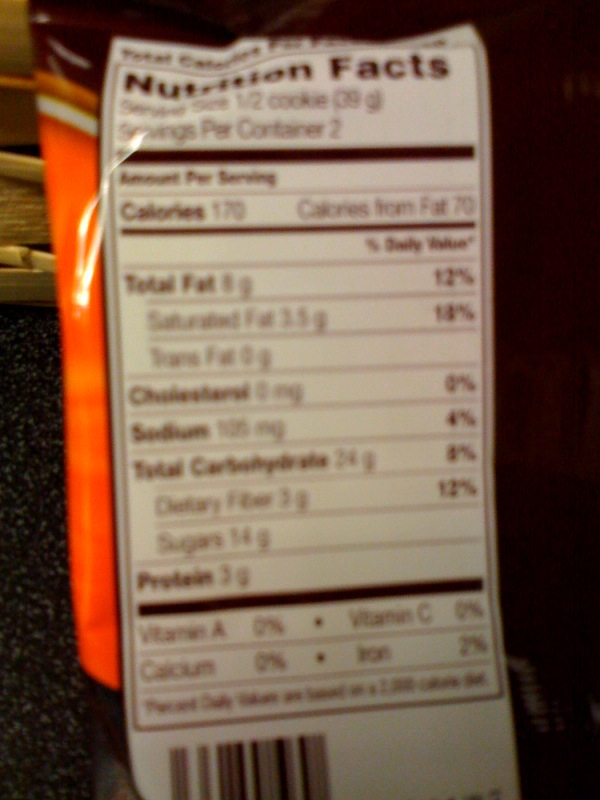A slightly blurry Nutrition Facts label is displayed against a vibrant red product bag. The white label with black text summarizes the nutritional content of the food item, which appears to be cookies. At the top, "Nutrition Facts" is clearly visible. The label ambiguously lists "12 cookies" and indicates a serving size of either 12 cookies or half a cookie, although the text is hard to decipher. It also states there are two servings per container. The number of calories is approximately 179, with 70 calories from fat. The label further details the amounts of total fat, cholesterol, sodium, total carbohydrates, and protein. Vitamins are minimal, reflecting the indulgent nature of the cookies, suggesting they are not the healthiest choice.